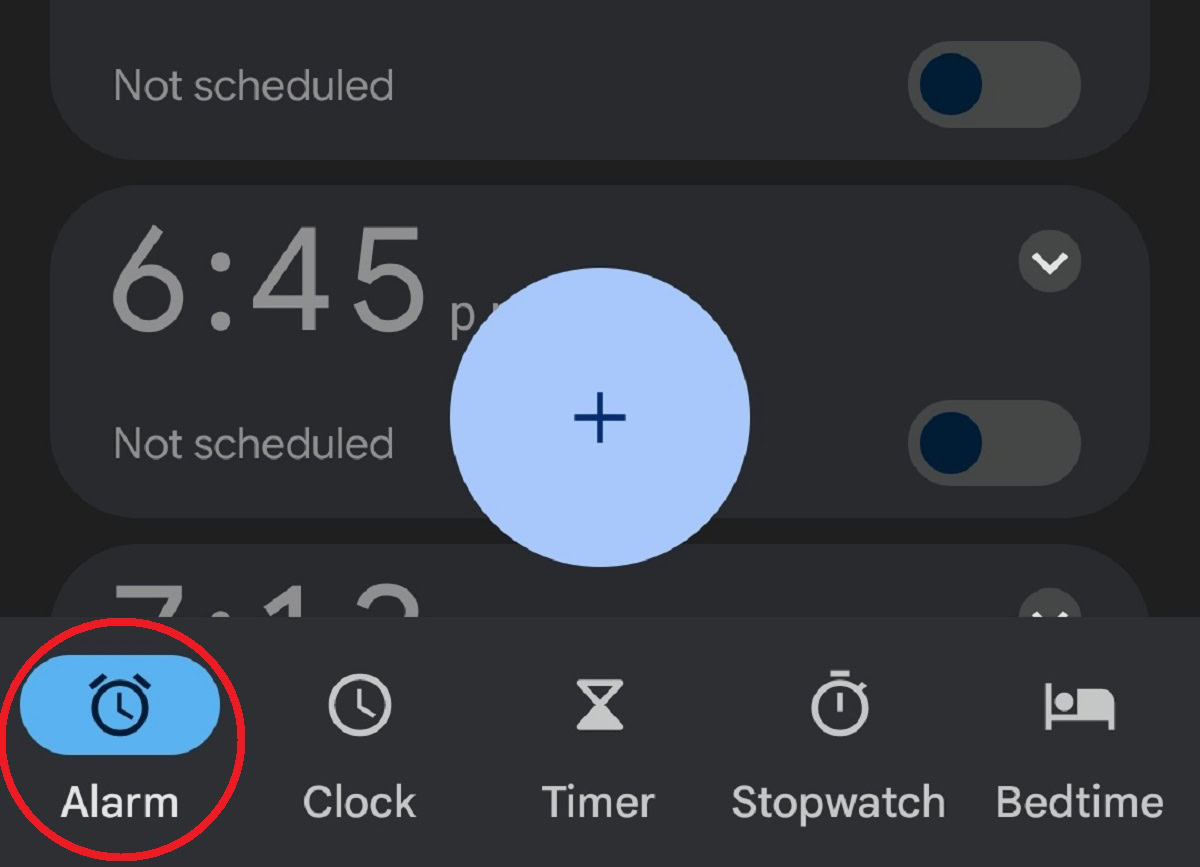This screenshot appears to be from a mobile app interface featuring a sleek night mode design with a charcoal gray background. At the top, there is a rounded-edged, lighter gray rectangle displaying the text "Not Scheduled" in gray font, accompanied by a toggle switch that is currently turned off. Below this component, a larger, lighter gray rectangle indicates "6:45 PM" in gray font, with "Not Scheduled" written below and a toggle switch that is also turned off. Superimposed above this section is a prominent sky-blue circle featuring a plus sign in the center, likely for adding new schedule entries.

Further down, partially visible is another rectangle showing a time, possibly "7:13 PM". At the very bottom of the image, the app's menu bar is visible, which includes the following options from left to right: "Alarm," "Clock," "Timer," "Stopwatch," and "Bedtime." Each menu item is paired with an icon; the "Alarm" option, which is circled in red, has an alarm clock icon, "Clock" features a clock icon, "Timer" includes an hourglass icon, "Stopwatch" displays a stopwatch icon, and "Bedtime" is represented by a bed icon.